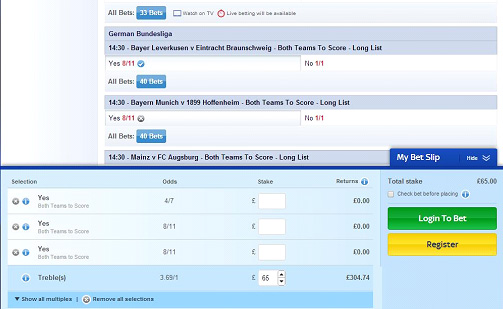This image is a screenshot from a sports betting website. On the far left side, there is a tall, thin, white rectangle. Just to the right of this rectangle, the page displays a section titled "All Bets," which currently shows a total of 33 bets. Below this, there is an option labeled "Watch on TV," accompanied by a clock icon, indicating the availability of live betting.

Prominently, the page features German Bundesliga match information: Bayer Leverkusen versus Eintracht Braunschweig scheduled for 14:30. The betting market for this match includes an option titled "Both Teams to Score - Long List" with the following odds: "Yes" is rated at 8/11, a selection that appears to be checked, while "No" is rated at 1/1.

Another match listed below also includes the "Both Teams to Score - Long List" option with identical odds of 8/11 for "Yes" and 1/1 for "No". This bet has accrued a total of 40 bets. The image not only provides current betting details but also highlights the website's user interface for placing live and pre-match bets on football games.